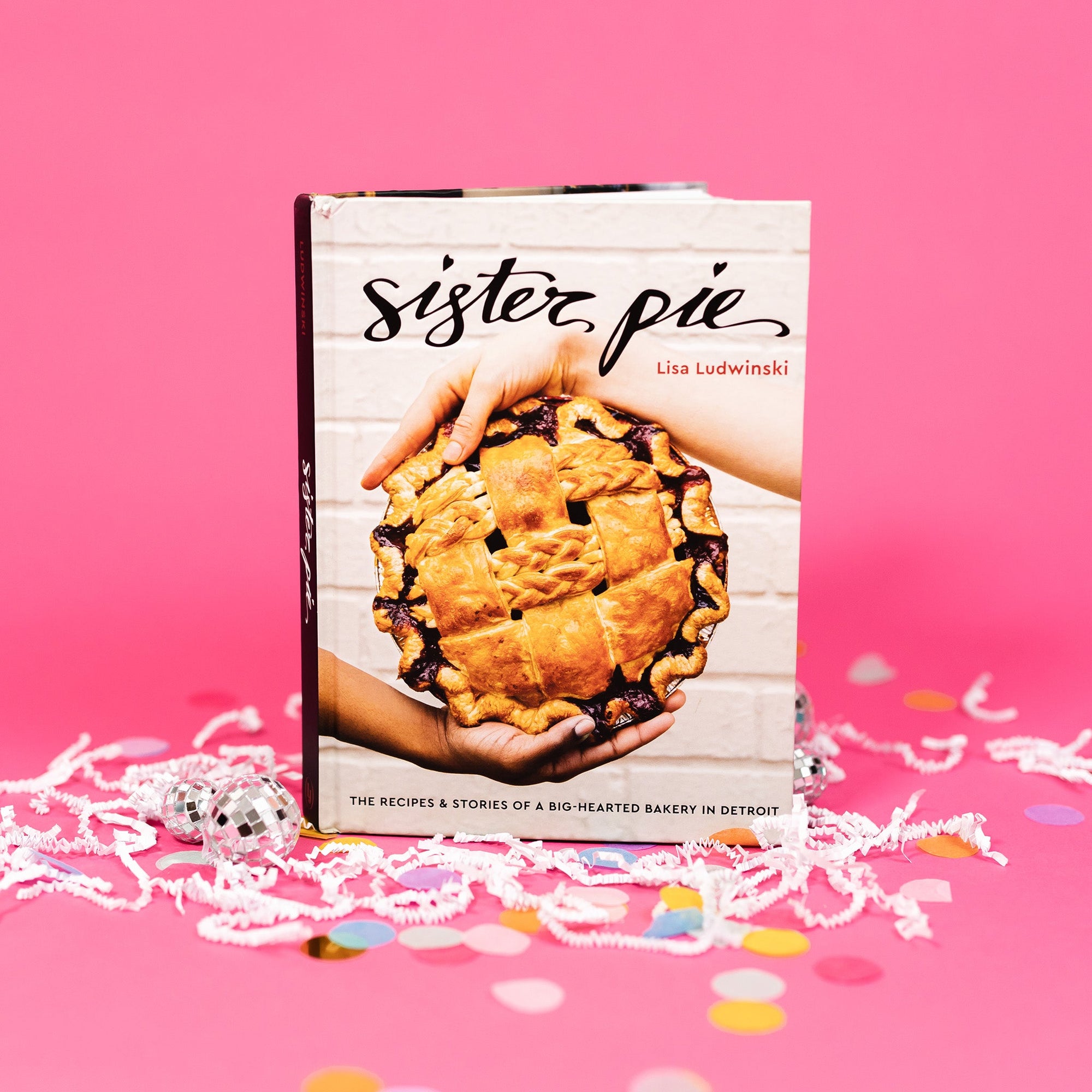This advertisement features the cookbook "Sister Pie" by Lisa Ludwinski set against a vibrant pink background. The focal point is the book itself, which stands prominently amidst an array of playful party decorations including colorful confetti and small glittery disco balls. The book cover showcases a lattice-crusted pie held by two hands—one fair-skinned hand on top and a brown-skinned hand on the bottom—symbolizing unity and community that the title "Sister Pie" evokes. The background behind the hands holding the pie is a white brick wall, and the title "Sister Pie" is written in all lowercase cursive. Beneath the pie image is the subtitle, "The recipes and stories of a big-hearted bakery in Detroit," highlighting the heartwarming and inclusive spirit of the bakery and the book. This festive setting suggests that the book can bring a sense of celebration and joy, much like a party.